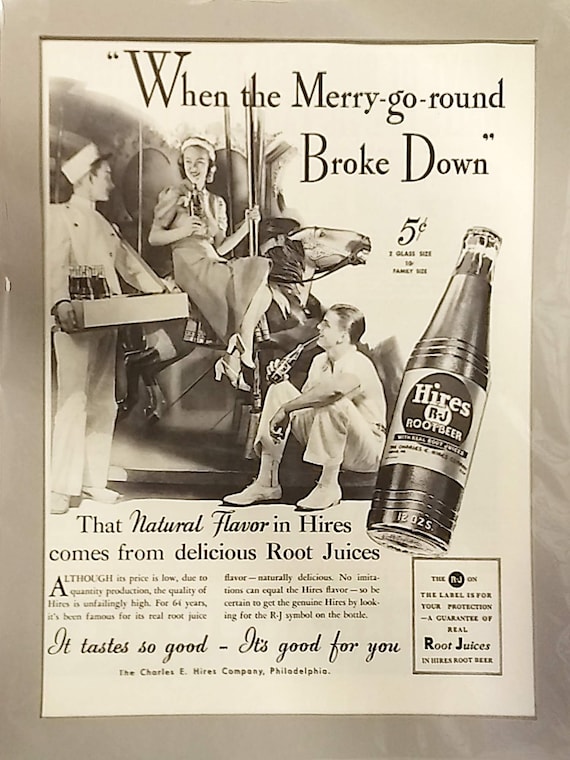This black and white or sepia-toned vintage poster, likely from the 1950s, is encased in a silver-colored frame and advertises 5-Cent Hire's RJ Root Beer, referencing "When the Merry-Go-Round Broke Down." The scene is set with a woman seated on a carousel horse, adorned in a dress, white heels, and a white headband. She holds a bottle of root beer in one hand while clasping the carousel pole with the other. Around her are two men: one dressed in a white usher's outfit and hat, carrying a tray with bottles of root beer; the other, on the actual carousel ring, sipping the root beer through a straw, flaunting slicked-back hair and light-colored attire. The bottle prominently features a metal cap and the label "Hires RJ." The poster boasts slogans such as "The natural flavor from Hire's comes from delicious root juices," and "It tastes so good. It's good for you." Additionally, a larger-than-life depiction of the root beer bottle is illustrated on the right side of the poster.